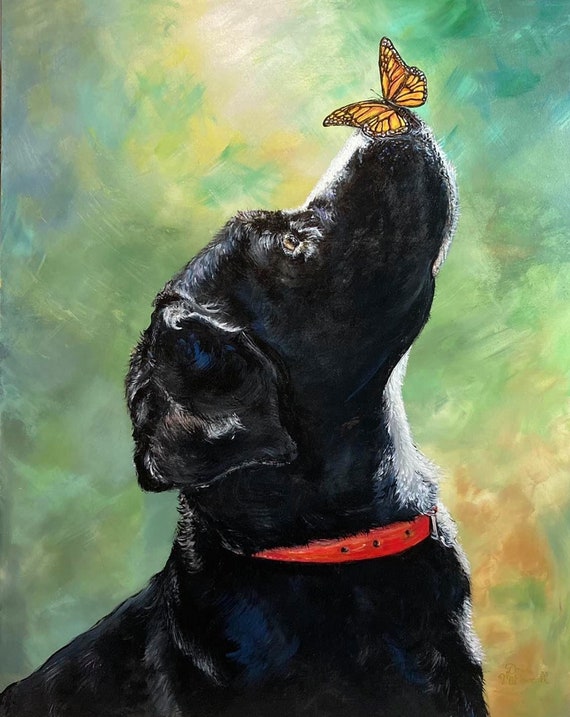This piece, which appears to be a painting or watercolor, vividly captures the scene of a black dog adorned with a red collar, prominently positioned in the vertical rectangular frame. The dog, possibly a black lab, occupies the center of the image, tilting its head upward and slightly to the right, showcasing its dark eyes and one visible ear. Notably, a monarch butterfly rests delicately on the dog's nose, its wings spread, creating a striking focal point. The background is an abstract blend of green, gray, brown, with hints of yellow and white, painted to convey a blurred, swirling effect. This colorful backdrop also features a circular, sun-like shape just left of the center, adding a whimsical touch to the serene and curious demeanor of the dog as it gazes at the butterfly.